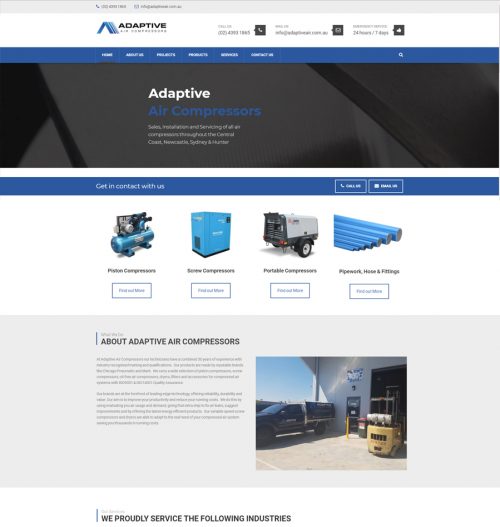This is a screenshot of a website named "Adaptive" that specializes in air compressors. At the top, there's a gray and white header featuring the company name "Adaptive" within it, indicating "Adaptive Air Compressors." This section also displays a phone number, an email address, and what appear to be business hours, though the details are somewhat difficult to read.

Below this header, there's a prominent black and blue banner. The black portion states "Adaptive Air Compressors," while additional text, somewhat blurry, appears beneath it. The blue part of the banner includes navigational options, where "Home" and "About Us" are readable, followed by a "Contact Us" button on the right. Other navigation items remain unclear.

Further down, there's a section encouraging contact, featuring a box labeled "Call and Email." Displayed below this banner are various images representing their product offerings: "Piston Compressors," an indistinct box, "Portable Compressors," and "Pipe Work, Hose, and Fittings."

At the bottom of the screen, there's a segment titled "About Adaptive Air Compressors," accompanied by a photograph of their workspace, which shows the exterior of a building, a truck, and some equipment.